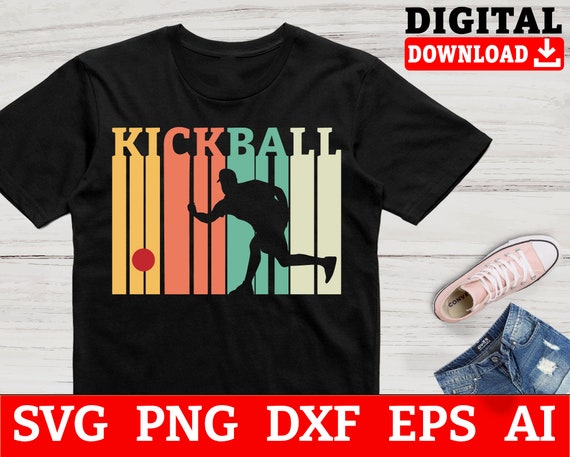The image is a digital mock-up of an advertisement for a black short sleeve t-shirt prominently positioned in the center. The shirt features the word "kickball" across the chest, with each letter extending downward like drips of paint. The colors of the letters are as follows: "K" and "I" are yellow, "C" and "K" are pink, "B" and "A" are green, and "L" and "L" are white. Inside these drips, there is a silhouette of a man in black, appearing to throw a red ball, located to the right of the letters. In the upper right corner, the word "DIGITAL" is written in black font above the word "DOWNLOAD" in white font on a red rectangle, accented with a white downward arrow. On the right side of the t-shirt, there's a pink tennis shoe over a pair of blue jean shorts. The bottom of the image features a red banner with large white text displaying the file formats available: "SVG", "PNG", "DXF", "EPS", and "AI." The items are arranged on a light-colored wooden surface with horizontal planks, adding a rustic backdrop to the display.